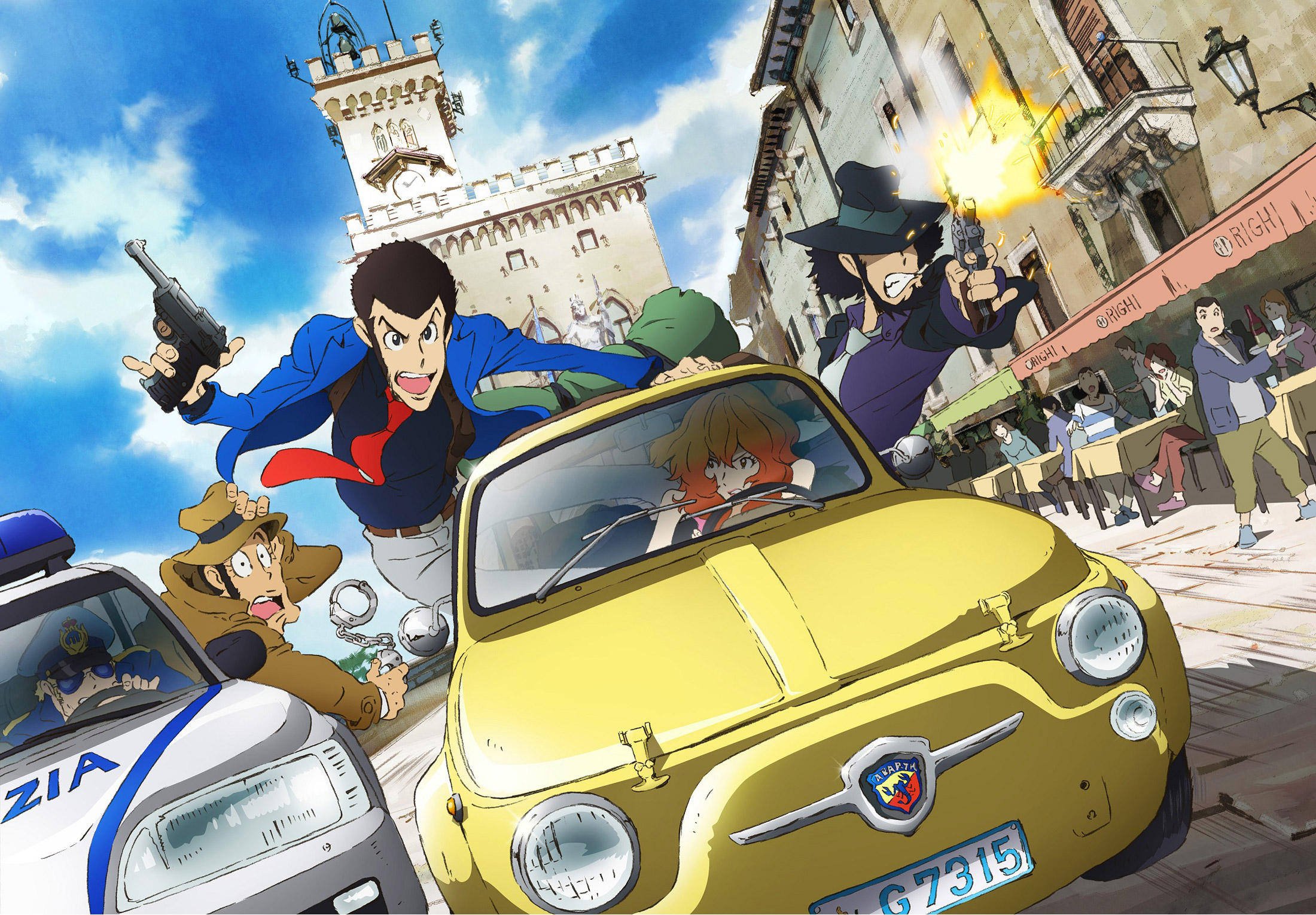This vividly animated frame appears to be from a Japanese-style anime during an intense car chase. The scene centers on a yellow-gold car, driven by a red-haired woman, hurtling through an old European city. There are two men brandishing guns out of the car's windows. The man on the passenger side, with slick black hair, is dressed in gray slacks, a dark blue shirt, a solid red tie, and a lighter blue sports coat; he appears to be shouting with his mouth wide open, his sharp triangular eyebrows raised in urgency. The other man, leaning out of the driver’s side window, wears a navy shirt and gray tie, paired with a gray fedora hat accented with a green-gray band, and is actively firing his gun, indicated by the bright yellow muzzle flash.

In hot pursuit is a white police car, visible at the bottom left of the frame. The detective, wearing a cliché noir-style brown trench coat and a similar brown hat, is seen hanging out of the back, sporting an expression of exasperation with wide eyes and an open mouth. He holds handcuffs in his right hand while steadying his hat with his left. The uniformed police officer driving the car is mostly hidden; only his sunglasses are visible, giving him a distinctly intense look as he maneuvers the vehicle close to the yellow car. The white police car, marked with the license plate GS315 and featuring a blue light on top, threatens to collide with the yellow car.

The setting is richly detailed, featuring Italian or French-inspired architecture with old stone buildings and a bustling street-side café on the right, where alarmed patrons sit under a bright red awning. A clock tower rises in the background against a blue sky scattered with a few clouds, adding to the lively, yet perilous atmosphere of this daytime chase.